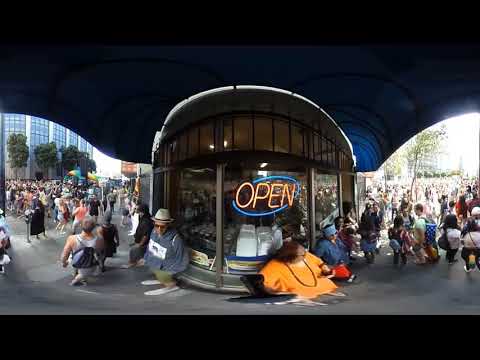The image depicts a bustling urban environment centered around a store with a large glass window and a conspicuous neon "OPEN" sign featuring orange lettering within a blue circle. The store is sheltered by a canopy, creating a shaded area amidst a sea of people who crowd the street and sidewalk around it. To the left and right of the canopy, the scene opens up to bright sunlight, revealing tall buildings with blue windows, some adorned with green trees. The crowd is diverse, consisting of both standing and seated individuals, including a notable woman in an orange outfit prominently positioned near the neon sign. The bottom of the image shows some distortion, but a man in sunglasses, a hat, a blue shirt, and white shoes can be discerned. This lively tableau suggests the setting of a festival, parade, or an exceptionally busy shopping district in a large city.